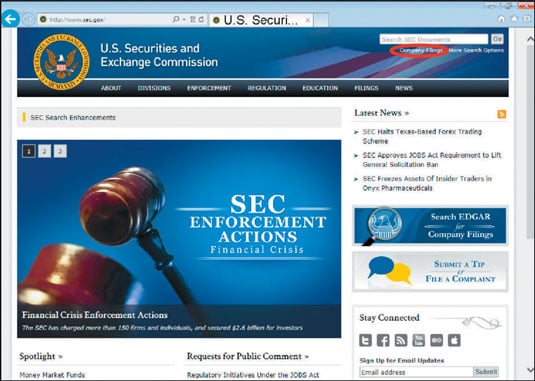This is a detailed screenshot of the U.S. Securities and Exchange Commission (SEC) website. The homepage features a structured layout with various sections and functionalities aimed at providing comprehensive information and resources. The top section prominently displays the SEC logo, establishing authenticity and official status.

The website navigation bar includes distinct categories such as Divisions, Regulations, Education, and News, ensuring easy access to specific information. A notable feature is the SEC Search Enhancement tool positioned on the right-hand side for refined searches.

Highlighted in the Latest News section are three significant updates:
1. SEC halts Texas-based Vortex trading scheme.
2. SEC approves implementation of the JOBS Act requirement, lifting the ban on general solicitation.
3. SEC freezes assets of insider traders in Onyx Pharmaceuticals.

Further down, options are available for users to search the EDGAR database for company filings and to submit tips or file complaints. There is also a "Stay Connected" box for visitors to subscribe to email updates.

The Spotlight section focuses on Money Market Funds and invites public comments on regulatory initiatives under the JOBS Act.

Overall, the site is a comprehensive resource with clear branding and user-centric features aimed at enhancing public engagement and regulatory transparency.